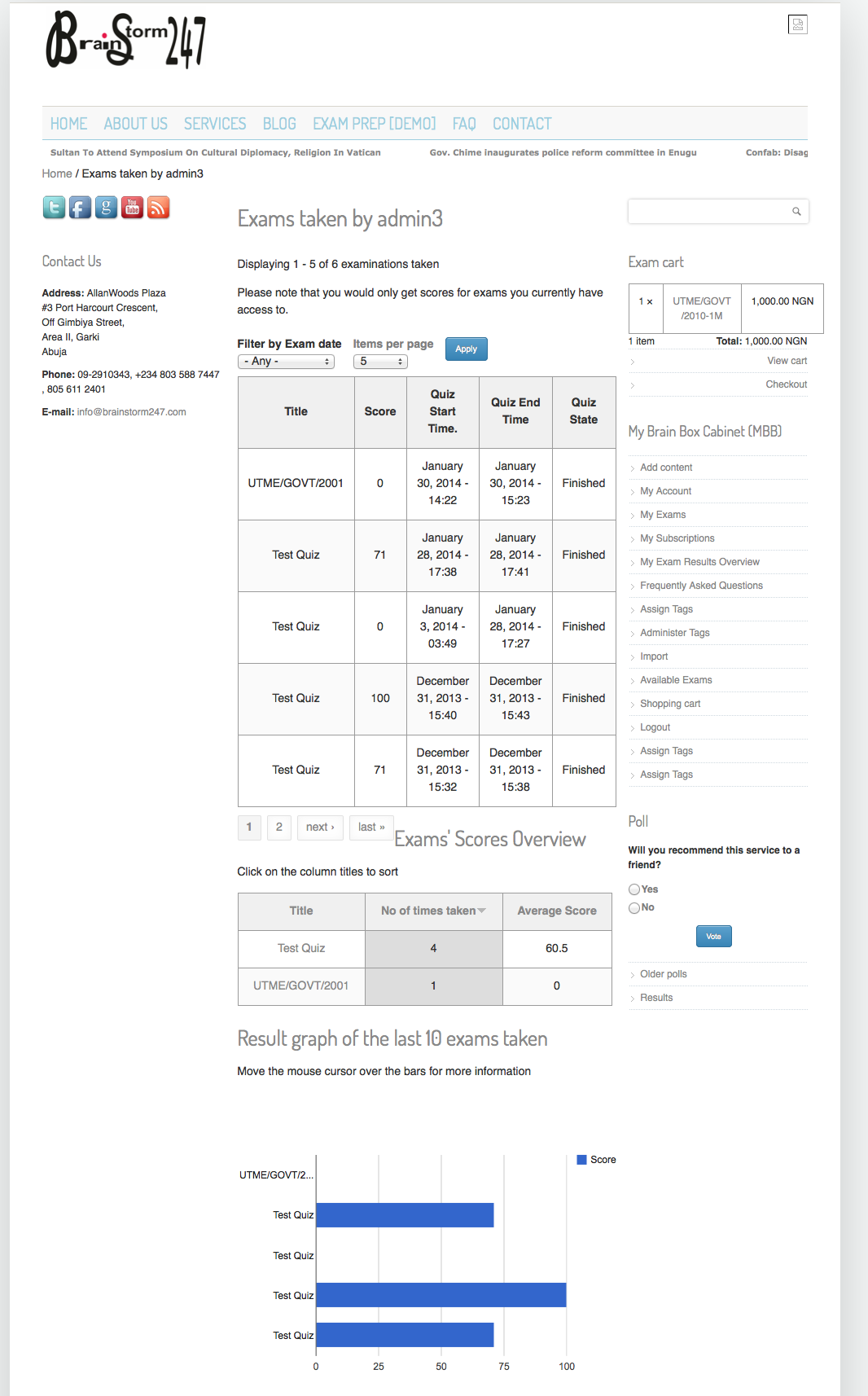The image appears to be a partial screenshot of a webpage, likely taken from a smartphone, displaying roughly three-quarters of the total page. Dominating the left-hand side, there's a heading that reads "Brian Brainstorm," written predominantly in cursive font, particularly emphasized on the 's' characters. This is followed by the numbers "24" and "7" positioned closely together without any separation, indicating "24/7" service.

On the right-hand side, there's a box-like element which contains indiscernible content. Below this box, a horizontal banner features a navigation menu with the following options: Home, About Us, Services, Blog, Exam Prep, Demo, Back, and Contact. 

Underneath the navigation menu, there is some line-separated information, accompanied by social media icons. Further down, details about contact methods are displayed under a "Contact Us" section. Next, there's a segment tagged "Exams Taken by Admin: 3," presenting data such as "Displaying 1-5 of 8."

Additionally, there is a notification stating: "Please note that you will only get access to exams you currently have access to." Below this, a filtered area organizes information into rows, with approximately six rows visible. Each row contains columns titled: Title, Score, Quiz Start Time, Quiz End Time, and Quiz ID.

At the bottom of the image, a results graph is depicted, with the results represented in blue.